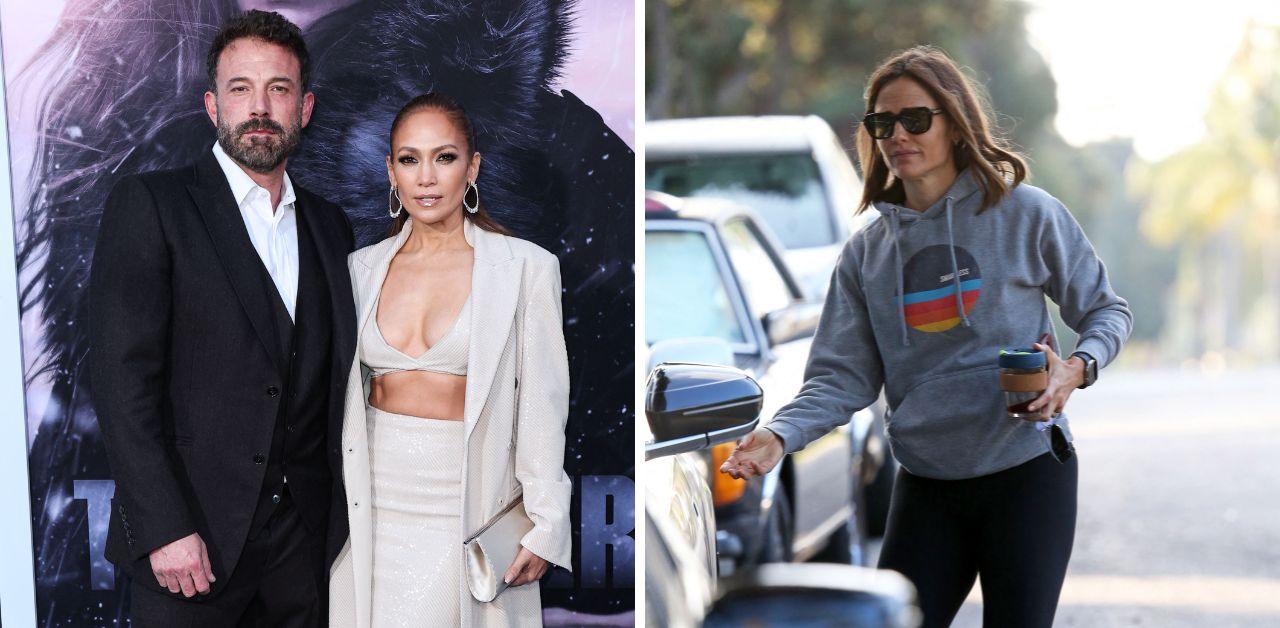In these side-by-side images, the photo on the left captures Ben Affleck and Jennifer Lopez, seemingly at a premiere event. Ben Affleck is dressed in a stylish black suit paired with a white collared shirt and an open vest. Beside him, Jennifer Lopez stuns in an all-white ensemble consisting of a long blazer jacket, a halter bralette top, a skirt, and a clutch purse. She accessorizes with large hoop earrings and has her hair pulled back in a sleek ponytail. Behind them, a partially visible poster, possibly depicting some kind of animal, adds to the event's atmosphere. On the right, Jennifer Garner, wearing a gray sweatshirt with a vibrant retro circle graphic featuring dark blue, light blue, red, orange, and yellow hues, appears to be getting ready to open a vehicle door. She is holding a clear glass cup and is dressed in black leggings and sunglasses, giving the impression of a casual, sunny day out.